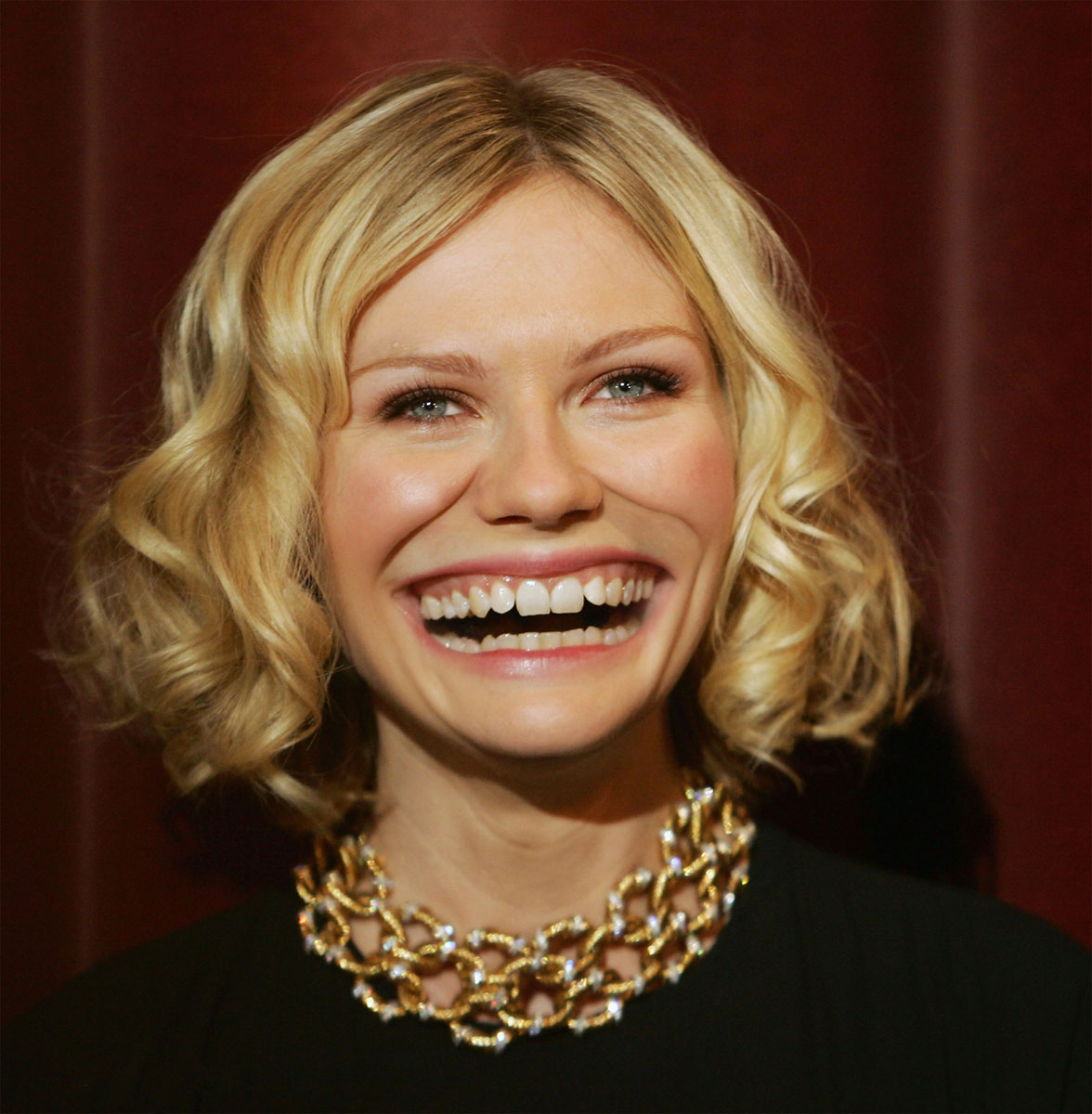This indoor photograph features a lady standing in front of a deep burgundy red curtain with vertical lines, suggesting the curtains are closed. The central focus is on the lady, who bears a striking resemblance to actress Kristen Wiig. She has blonde, curly hair that reaches neck level and is parted in the middle. Her blue eyes stand out prominently. She is dressed in a black garment, which could be either a dress or a top. Around her neck, she sports a thick, multi-row golden chain necklace with silver accents and white jewels. The image appears to be digitally altered, particularly in the area of her mouth, which is exaggeratedly wide and shows all her perfectly straight teeth, suggesting a heavy-handed use of photo editing. There is a slight shadow behind her, cast on the lower part of her hair, adding depth to the photo.